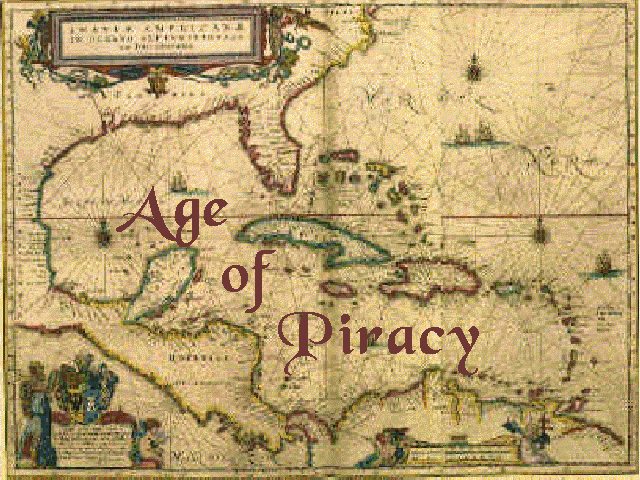The image depicts an aged-looking map designed to evoke the era of piracy, with a generally yellowish-brown patina to give it an antique feeling. At the center, in large maroon text, it prominently displays the title "Age of Piracy," with each word slightly indented from the one above, creating a tiered effect. Surrounding this text, the map shows an outline that seems to represent parts of the United States, including the recognizable shape of Florida, extending down toward Mexico and perhaps South America, though the exact regions are hard to discern.

In the upper left-hand corner, there is a rectangular box filled with text that appears too small and blurred to read. The map features a mix of yellow, maroon, and teal colors, enhancing its vintage appeal. Scattered throughout are pirate-themed illustrations, including pirates and little islands, and in the bottom left corner, there are depictions of people, possibly more pirates or figures dressed in period attire. The overall design and markings contribute to the impression that this is a historically styled map, perhaps illustrating a pirate's routes or territories during the "Age of Piracy."